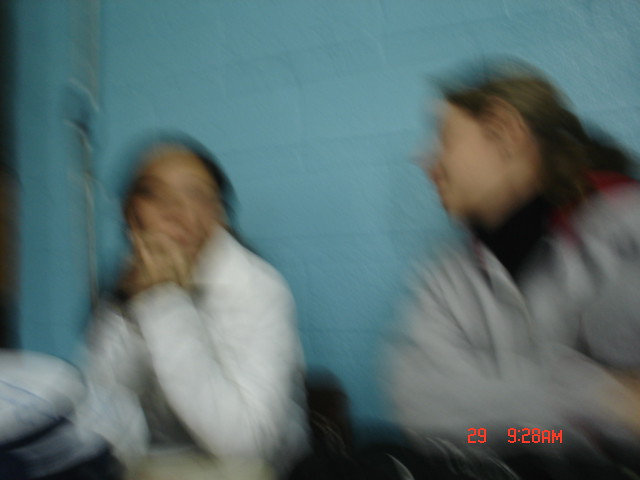A blurry still image captures a moment between two women seated in a small room with turquoise-painted cinder block walls. In the bottom corner, red text displays "29" and "9:28 a.m." On the left, a woman with dark skin and dark hair is dressed in a white jacket or long-sleeve shirt. Opposite her, on the right, sits a woman with a sallow complexion and brownish hair, wearing a gray jumper, sweater, or shirt. They appear to be engaged in a conversation, but the blur obscures additional details in the foreground.